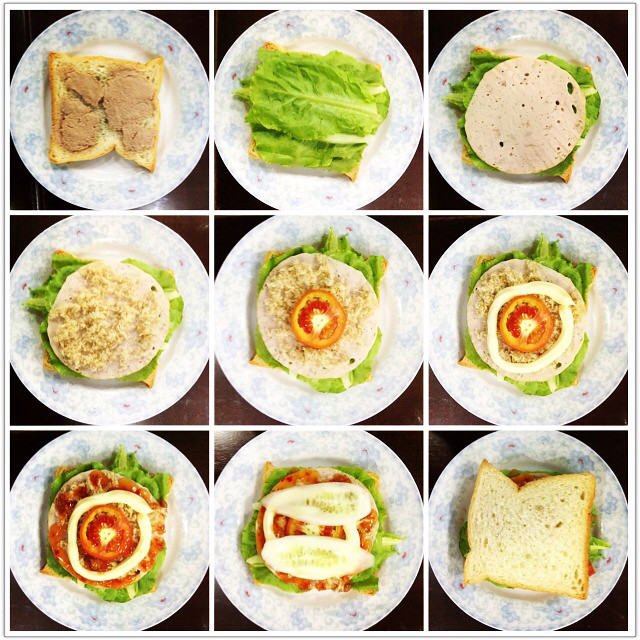The image displays a 3x3 grid of blue and white patterned plates, each illustrating different steps in assembling a sandwich. Starting from the top left, there's a slice of bread with roast beef, followed by a plate with just lettuce. Next to it is a plate with lettuce and ham. Moving down to the second row, the left plate adds a topping, possibly a tortilla-like wrap, to the sandwich. The middle plate includes a tomato slice and a white ring of sauce. The right plate shows a more detailed assembly with tomato and sauce. In the bottom row, the left plate starts with a slice of bread, lettuce, tomato, and a white ring, possibly onions or another topping. The middle plate adds cucumbers and sauce to the mix. Finally, the bottom right plate completes the sandwich with a top slice of bread, showing hints of green and red ingredients inside. This collage clearly depicts the detailed process of making a fully assembled sandwich.